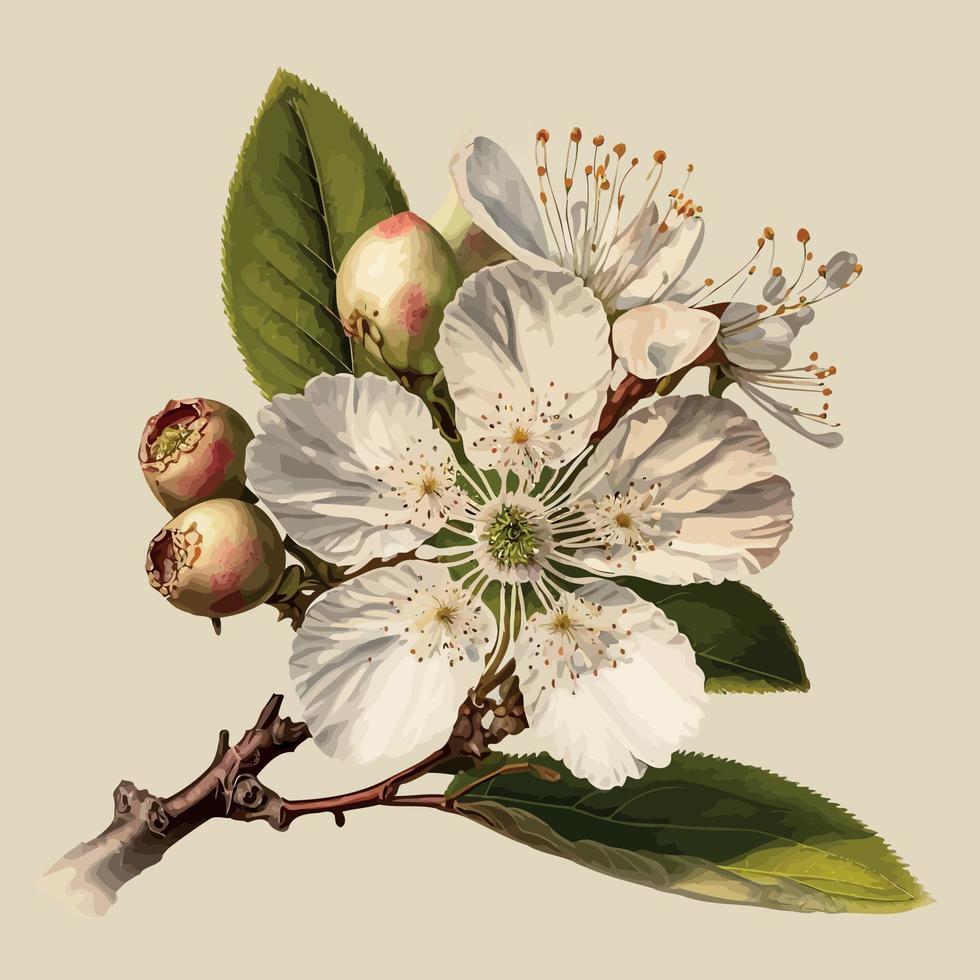This image is a detailed drawing of a flower, likely created using digital or acrylic painting on a sheet of beige-colored paper. The image is square, with equal lengths for all four sides, and features a tan solid color background. 

At the center of the artwork is a thick, dark brown tree stem that branches out into lighter, more reddish stems. These stems then further branch into intricate leaves and flowers. The leaves are oval-shaped with small ridges along their edges and light white veins running through them. Additionally, the drawing includes berry-like plants that are red and white with green-tipped openings.

The central flower prominently features five white petals surrounding a green center. Each petal contains smaller, seed-like elements with dots around them, adding to the complexity of the design. There are at least two other flowers depicted, although their petal counts are less clear as they face different directions. The illustration also includes three leaves growing from a single branch, each with spiked edges, and forms part of a highly detailed botanical piece.